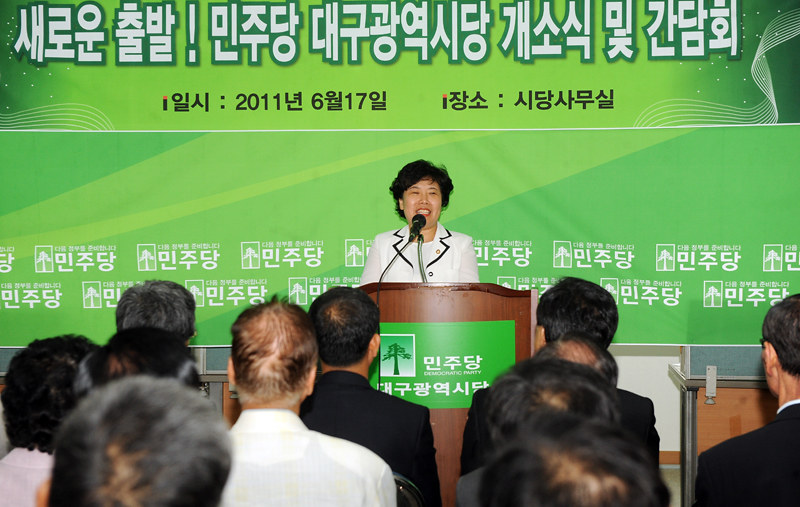The image portrays an Asian woman, approximately 45 years old, standing and speaking at a business conference. She is positioned behind a wooden podium and speaking into a microphone, with a warm smile on her face. The woman has short black hair that falls to her ears and is dressed in a white business jacket, distinguished by black pinstripes on the collar and brass buttons. The podium displays a green sign adorned with a bonsai tree logo and Chinese writing. Behind her is a bright, neon green billboard also featuring white Chinese characters prominently at the top, with additional black text and a date: 2011.6.17, presumably indicating the event date. The audience consists of eleven people—all seated with their backs turned to the camera—majorly men, with at least two donning white shirts and a few in black jackets. The setting suggests a formal setting or a business conference with significant emphasis on presentations or discussions.